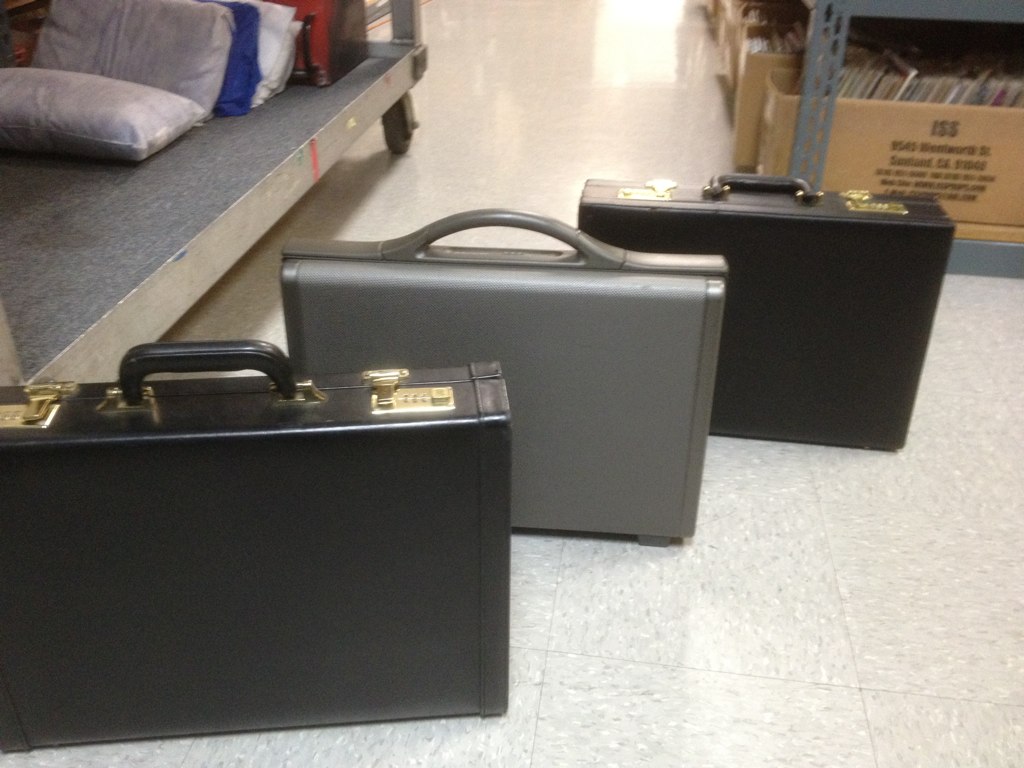This detailed photograph captures a floor-level view showcasing three medium-sized briefcases standing upright on a highly reflective, white vinyl tile floor, buffed to a shine. The briefcases are positioned between a metal cart on the left and a gray metal rack on the right. The closest briefcase is black with gold combination locks and a handle. Behind it is a gray briefcase with a matching handle, devoid of any locks or additional features. The third briefcase at the back mirrors the black one at the front, also featuring gold combination locks. 

To the left of the briefcases, there is a metal cart with open sides and rails at the ends, holding a red box along with white and blue pillows. On the right side, the bottom level of a metal shelf rack is partially visible, supporting cardboard boxes that appear to contain books. The reflective floor hints at overhead lighting, placed outside the image's edges, contributing to the overall illumination of the scene.